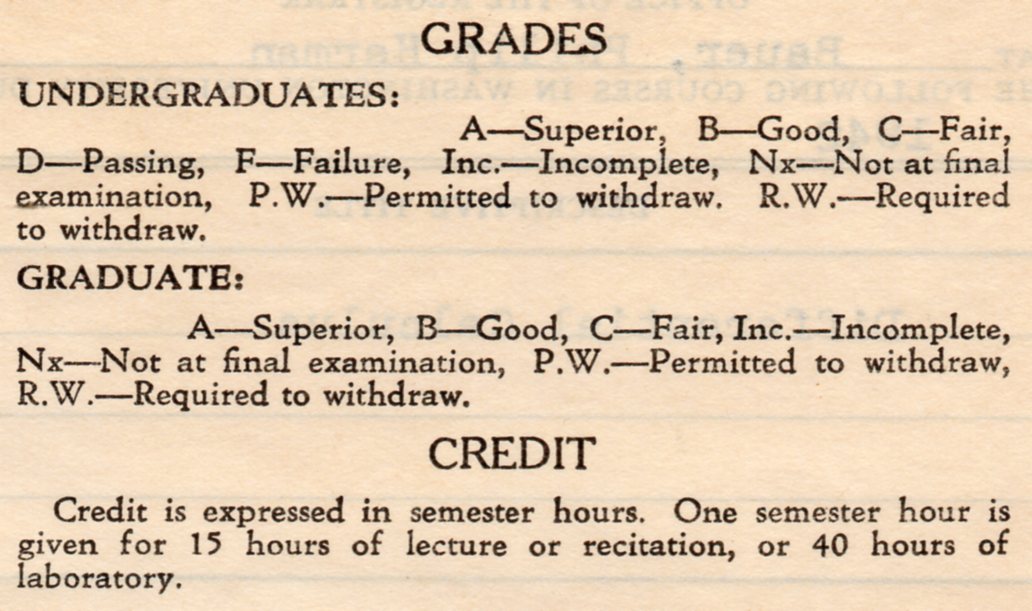The image depicts an old university or school document, probably a student handbook, detailing the grading and credit system. The title of the paper is "Grades," and it describes grade classifications for both undergraduate and graduate students in black text arranged in three rows with subheadings. For undergraduates, the grades are listed as follows: A (Superior), B (Good), C (Fair), D (Passing), F (Failure), Inc (Incomplete), Nx (Not at Final Examination), Pw (Permitted to Withdraw), and Rw (Required to Withdraw). For graduate students, the grading is similar but without a grade D: A (Superior), B (Good), C (Fair), Inc (Incomplete), Nx (Not at Final Examination), Pw (Permitted to Withdraw), and Rw (Required to Withdraw). The document describes the credit system, explaining that one semester hour is awarded for 15 hours of lecture or recitation, or 40 hours of laboratory work. The paper is brown, suggesting its age, and the text is printed in a classic font style, reinforcing its old-school appearance.